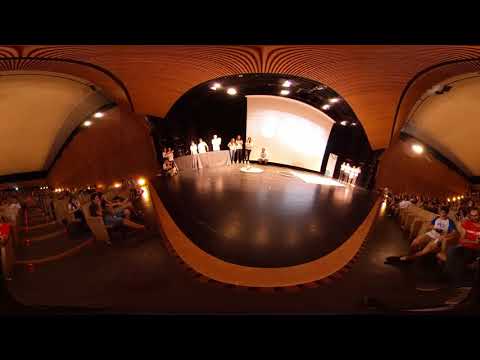This is a wide-angle photograph, somewhat manipulated to appear overly curved and round, capturing a dramatic scene in an auditorium. Centrally, several people wearing white tops stand and perform on a dark brown or black stage, which is framed by a rich, lighter brown wooden base. A prominent white screen hangs behind them, illuminated by bright, circular lights from the reddish-orange ceiling. To both the left and right, a scattered audience sits, with many visible feet protruding into the aisles, although not all seats are occupied. The setting features stairwells on the sides ascending to the top of the auditorium, accentuating the room's darker ambiance. Despite the distortion, it’s evident that the event is theatrical and set in a classic auditorium with well-defined lighting.